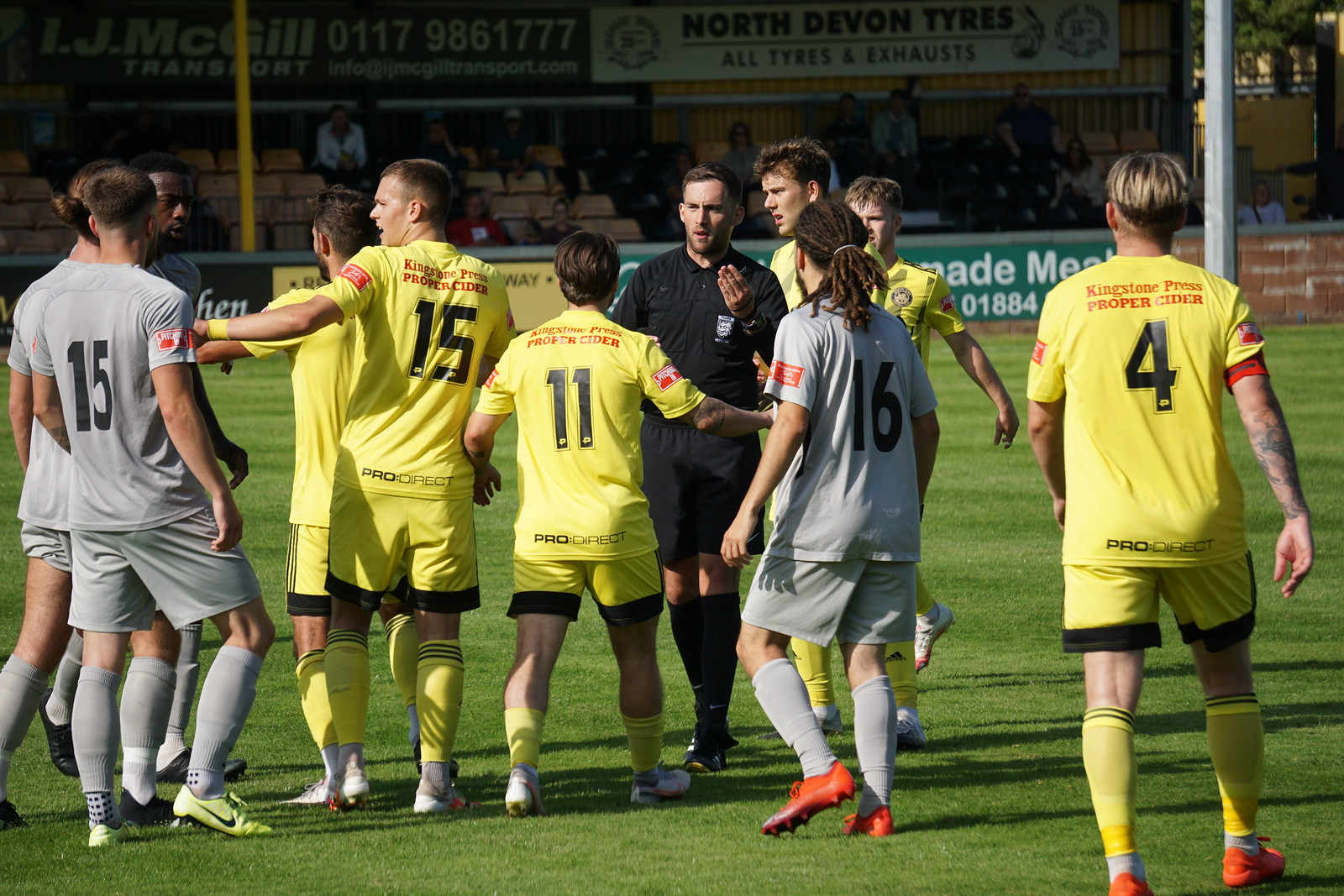The photograph captures a tense moment on a soccer field with a group of young male players from two teams gathered around a central figure dressed in black, likely a referee. The teams are distinguishable by their uniforms: one team wears yellow jerseys with black trim, yellow shorts, and socks, branded with "Kingstone Press Proper Cider" on the back, while the other team sports gray jerseys, shorts, and socks with only numbers on the back. On the green field, a player in a yellow uniform with outstretched arms appears to be touching the chest of a gray-uniformed player, suggesting a heated exchange. The referee, positioned in the center and facing the camera, seems to be intervening in the potential confrontation. In the background, there are spectators in the stands and advertisement banners, including ones for "T.J. McGill" and "North Devon Tires, All Tires and Exhausts."